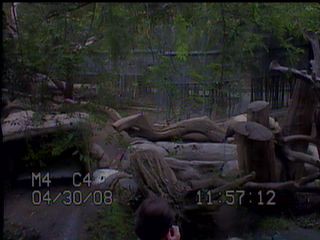This image is a small, rectangular, and very dark outdoor photograph that appears almost as a video still. Dominated by shades of black, green, and brown, it depicts a mysterious scene reminiscent of a swamp or a zoo at night. In the background, a dense thicket of closely packed trees, branches, and leaves is visible. The faint reflection of houses can be seen on the very still water. In the top right corner, darker tree trunks are discernible amongst more greenery. The largest element in the foreground is a curved log or fence-like structure made up of haphazardly stacked, dull brown logs. Additionally, there are rocks on the left and potentially the back of someone's head and hand, possibly capturing a photo, in the bottom center. The image has a digital timestamp reading "M4 C4 04/30/08 11:57:12" at the bottom right, adding to its cryptic nature.